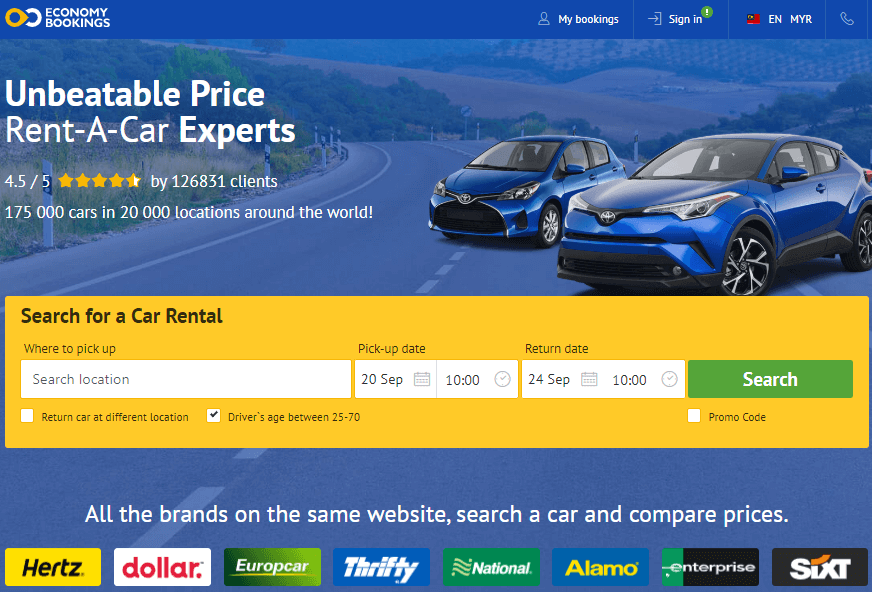The image features a detailed advertisement for a car rental service on a blue background. At the top, there's an orange logo resembling an "O" with a point, next to a double-headed white arrow. The text "Economy Bookings" is prominently displayed. Below it, there are options for "My Bookings" and a "Sign In" button housed within a box, featuring a right-facing arrow.

Further down, a green circle with an exclamation point and a red box containing a black and yellow icon can be seen. The text "EN" (likely indicating the language) and "MYR" (possibly the currency) are shown next to a phone icon.

The centerpiece of the image showcases two stunning blue cars parked by the roadside. Text below highlights the service's promise with the phrases: "Unbeatable Price," "Rent-a-Car Experts," "4.5 out of 5 stars by 126,831 clients," and "175,000 cars in 20,000 locations around the world."

A prominent yellow box invites users to "Search for a Car Rental." Fields are provided for location, pick-up date (20th September at 10:00 AM), and return date (24th September at 10:00 AM). A large green "Search" button is ready for action. Additional amenities include options for returning the car at a different location, a checkbox for drivers aged between 25 and 70, and a field for a promo code.

Towards the bottom, a notable blue box emphasizes, "All the brands on the same website," encouraging users to "Search a Car and Compare Prices," with logos of popular car rental companies like Hertz, Dollar, Europe Car, Thrifty, National, Alamo, Enterprise, and Sixt arrayed below.